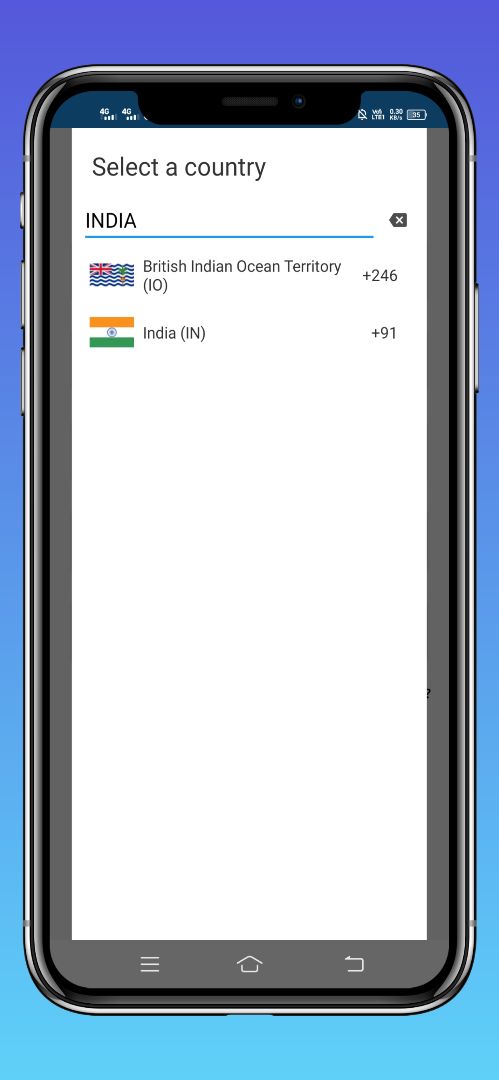This color image is rectangular in shape with its longer side oriented vertically. The background of the image transitions smoothly from a deep purple at the top, fading into a darker blue, and finally merging into a light sky blue at the bottom. A central element of the image is a profile view of a smartphone. 

Displayed on the screen of the smartphone is an interface featuring a predominantly blue background. At the top, in bold black text, are the words "Select a Country." Below this header, "INDIA" is written in all caps and underlined with a light blue line. To the right of the word "INDIA," there is an icon resembling a rectangular button containing a white 'X' and an arrow pointing to the left.

Beneath this blue bar, there are two entries featuring flags and corresponding country codes. The first entry displays the flag of the British Indian Ocean Territory, followed by the text in parentheses "(IO)," and to the right, the country code "+246." Below this, the second entry shows the flag of India, followed by the text in parentheses "(IN)," and to the right, the country code "+91."